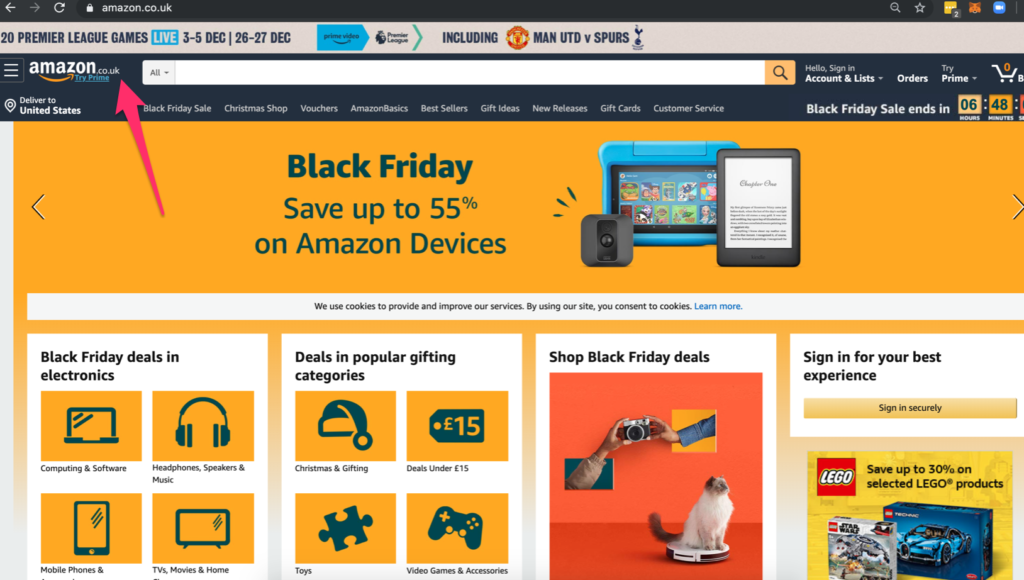The image is an Amazon Black Friday advertisement prominently featuring a large, elongated orange box with the text "Black Friday" in bold black letters. The ad highlights a promotion where customers can save up to 55% on Amazon devices. Included in the ad are images of several devices, notably a blue children's computer alongside two other gadgets.

A distinctive red arrow is pointing toward the word "Amazon," ensuring viewers recognize the brand. At the top of the ad, there is a search bar where users can type in queries, and just below this is a gray navigation bar with various clickable options, including an item labeled "Premier League Games."

Beneath the extensive orange box, additional Black Friday deals in electronics are displayed, with four images aligned on the left. Adjacent to this section, another part of the ad directs attention to "popular gifting categories," showcasing four more deals.

A significantly larger section with a black background emphatically encourages customers to "Shop Black Friday deals." This section is creatively illustrated with a quirky image of a cat riding a robotic vacuum and a photo of two hands holding a camera.

The ad also includes a reminder to users to "sign in for your best experience." Toward the bottom of the visual, there is a promotion for Legos, featuring two boxes prominently displaying the recognizable red Lego logo.